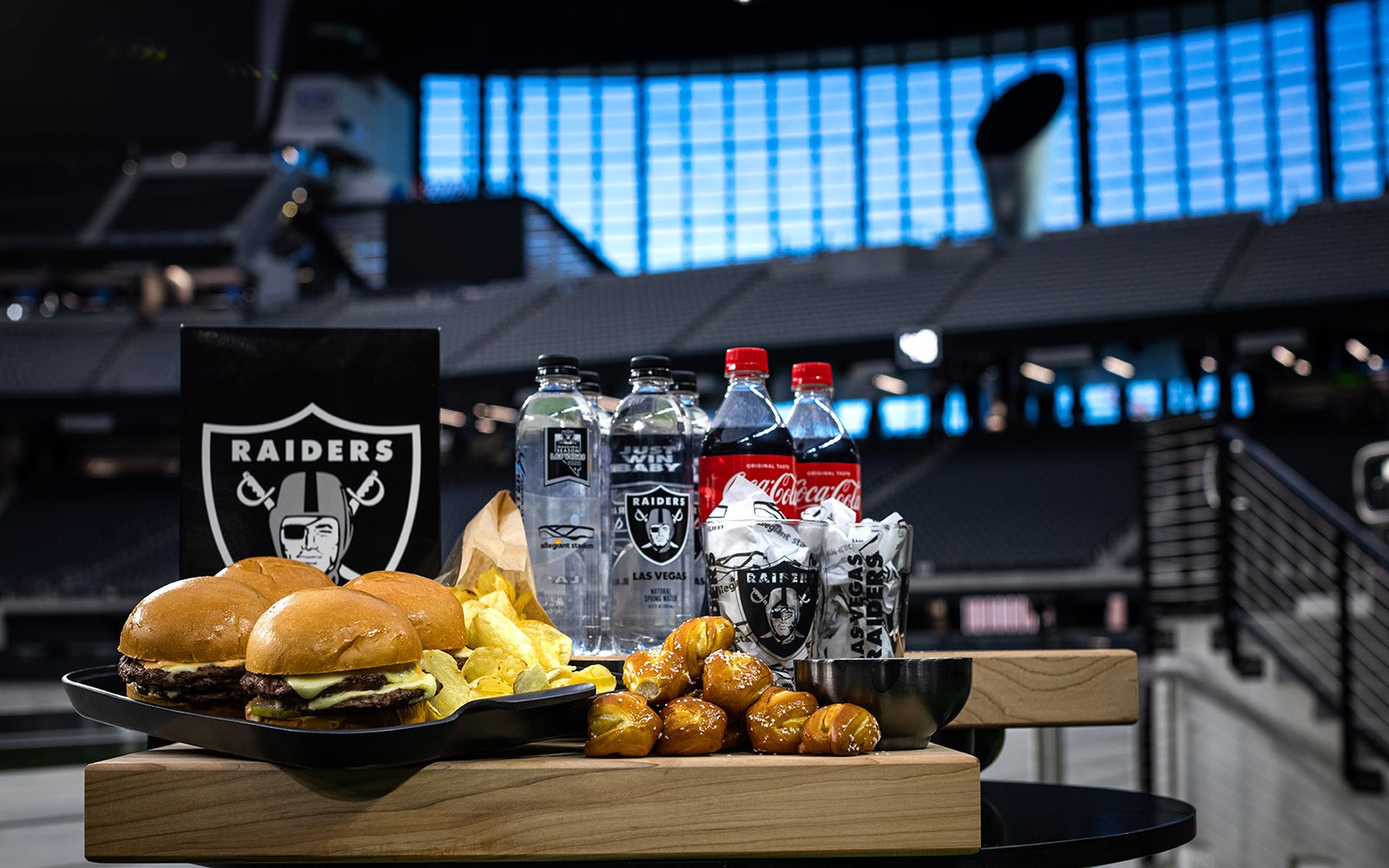In the image, a spread of food and drinks is artfully arranged on two wooden bases placed on a black table inside a large sports stadium. Dominating the center of the wooden bases is a black tray holding four fluffy brown cheeseburgers paired with crispy potato chips. To the right of this tray, a pile of seven salted pretzel bites is neatly arranged, next to a shiny dark bowl. In the background, elevated on a higher wooden platform, sit two bottles of Coca-Cola and two bottles of water, each branded with the Las Vegas Raiders logo. On the left center, there is a prominent black sign featuring the Las Vegas Raiders shield logo, showcasing a football player with swords behind his head. The backdrop consists of large blue sectioned windows and blurred stadium seats, tying in the atmosphere of a sports venue. A part of a staircase handrail is visible to the right of the setup, adding depth to the scene.